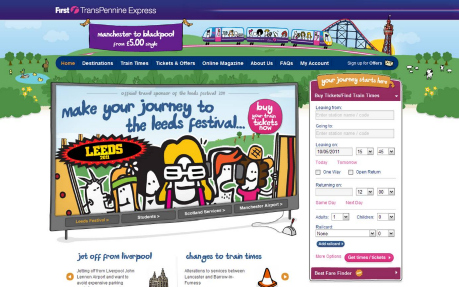This image showcases a promotional advertisement for First Transparency Express, highlighting their Manchester to Blackpool route with fares starting at just £5 for a single journey. The background displays a sleek, modern train in motion, emphasizing efficiency and speed. The advertisement features various categories including Home, Constructions, Train Times, Tickets and Offers, Online Magazine, About Us, Frequently Asked Questions, My Account, and Sign Up for Offers.

Notably, there are additional attractions mentioned such as "Make Your Journey to the Leeds Festival," and suggestions like "Buy Your Train Tickets Now." The advertisement further highlights seasonal events and travel opportunities, with prompts like "Leeds Yeti," "Jet Off from Liverpool," and "Changes to Train Times." The detailed and vibrant design of the advertisement encapsulates the convenience and excitement of train travel with First Transparency Express, appealing to potential travelers by emphasizing seasonal events, significant destinations, and ease of booking.